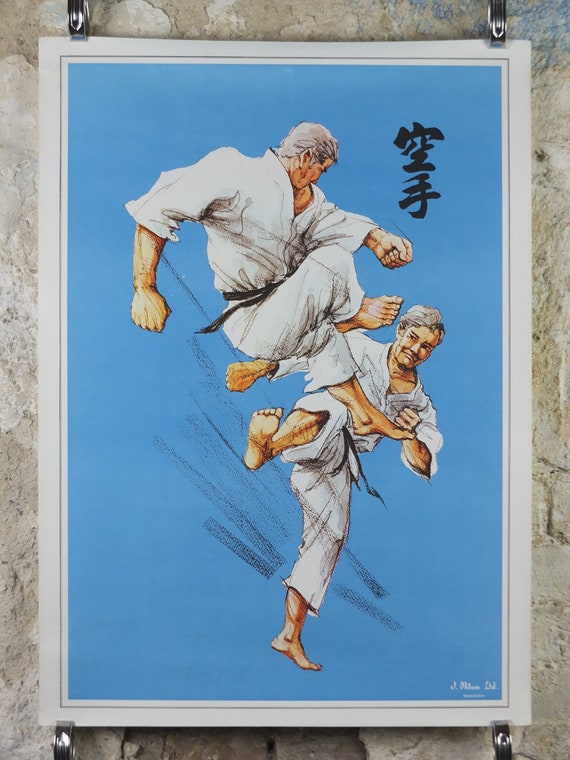The image is a detailed, color painting by Jay Milton, as indicated by his signature in the bottom right corner. This vibrant piece is bordered by a black line and set against a backdrop resembling a stone or rock pattern, similar to a kitchen counter tile. Dominating the scene is a dynamic depiction of two older men engaged in a martial arts battle, specifically karate, each dressed in white gi with black belts. One man leaps into the air, poised to deliver a head-kick, while the other attempts to block the attack on one leg. Their graying hair and focused expressions bring a sense of intensity and experience to the scene. Black streaks underscore the motion and energy of their combat against a solid blue background. At the top right corner of the painting, two Chinese or Japanese symbols add an element of authenticity and cultural context to the artwork.